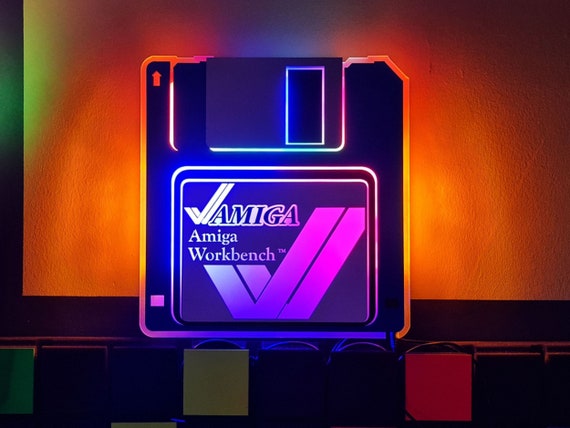The image features a retro floppy disk from the 90s, prominently centered against a vivid, neon-lit orange background. The floppy disk itself, characterized by a dark purple hue, exudes an iridescent rainbow sheen with vibrant outlines in purples, blues, oranges, and yellows. The label on the disk reads "Amiga Workbench," marked with a distinct double-tick logo. The logo and text are displayed on the area typically used for labeling file names. An orange arrow in the top right corner of the disk indicates the correct insertion direction. The entire scene evokes a nostalgic, retro-futuristic vibe reminiscent of the 80s and 90s, with a visual style akin to Blade Runner's neon aesthetics.